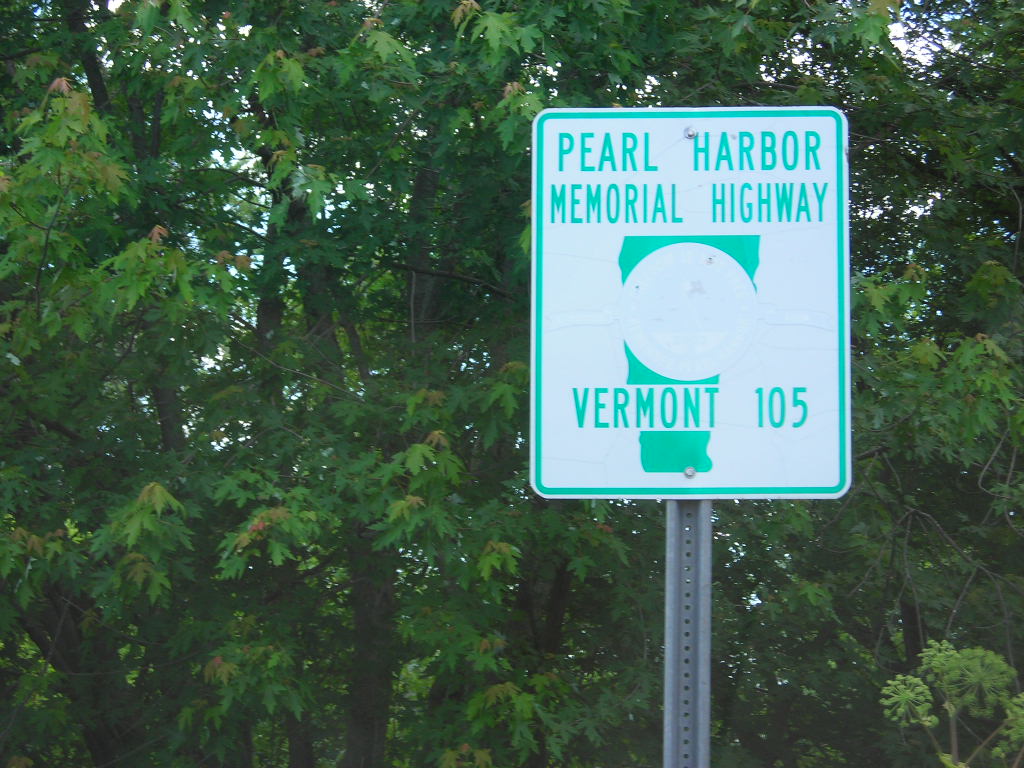The photo captures a detailed view of a street sign with the label "Pearl Harbor Memorial Highway," which designates Vermont Route 105. The sign is rectangular and predominantly colored in white with light green lettering. It features an emblematic outline of the state of Vermont with additional green accents on the top and bottom. This sign is mounted on a gray metal post perforated with numerous holes. The scene is set outdoors, amidst a lush background of closely clustered trees and bushes, displaying a vibrant mix of green foliage interspersed with occasional brown and yellow leaves. The tree trunks and branches peek through the foliage, with patches of sky visible in between.